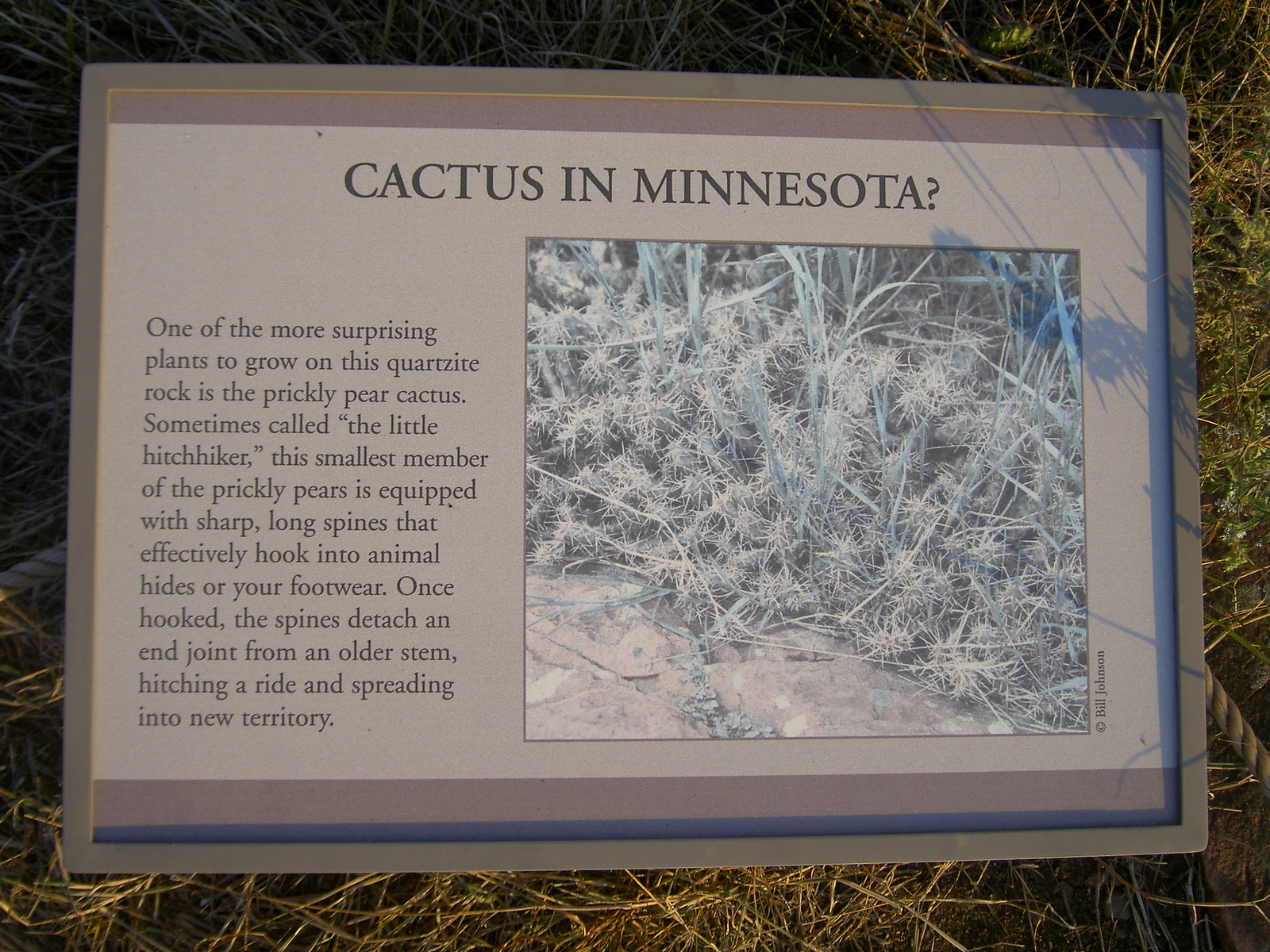The image depicts a photograph of a rectangular board framed in grey, placed on a patch of brown and green grass. The board features an article titled "Cactus in Minnesota." Positioned on the left side of the article is a detailed description of the prickly pear cactus, sometimes referred to as the Little Hedge Hiker or the little hitchhiker. This smallest member of the prickly pear cactus family is noteworthy for its long, sharp spines that can hook into animal hides or footwear, detach from the older stems, and spread to new territories. To the right of this informative text is a photograph of a cactus plant adorned with many spikes. The overall scene captures the unexpected growth of the prickly pear cactus on a quartzite rock, emphasizing its unique adaptation and spread.